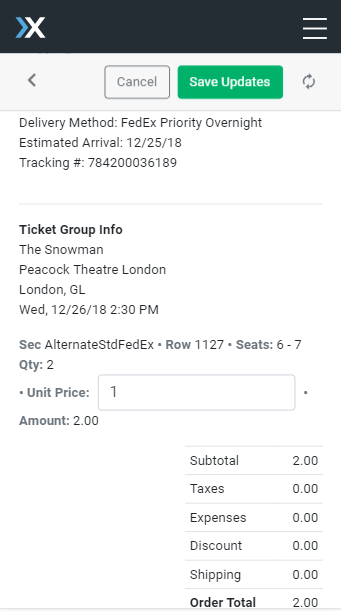**Caption:**

The website interfaces with a clean, modern design characterized by a black top bar featuring three horizontally-aligned lines on the left. Beneath this, a gray section includes a left-pointing arrow and several circles with arrows on the right side. A green bar labeled "Save Updates" and a lighter bar labeled "Cancel" are prominently displayed. 

The delivery method is listed as FedEx Priority Overnight with an estimated arrival date of 12-25-18, accompanied by a tracking number. The middle section details "Ticket Group Info," specifying an event "The Snowman" at the Peacock Theatre in London, GL on Wednesday, 12-26-18 at 2:30 PM. Alternate seating information includes Row 11-27, Seats 6-7. The ticket quantity is 2, priced at $1.00 each, totaling $2.00. The order summary shows a subtotal of $2.00, with no additional taxes, expenses, discounts, or shipping charges, resulting in an order total of $2.00. 

Overall, this section of the website provides users with detailed tracking and order information, along with an option to manage their ticket delivery if delays occur.